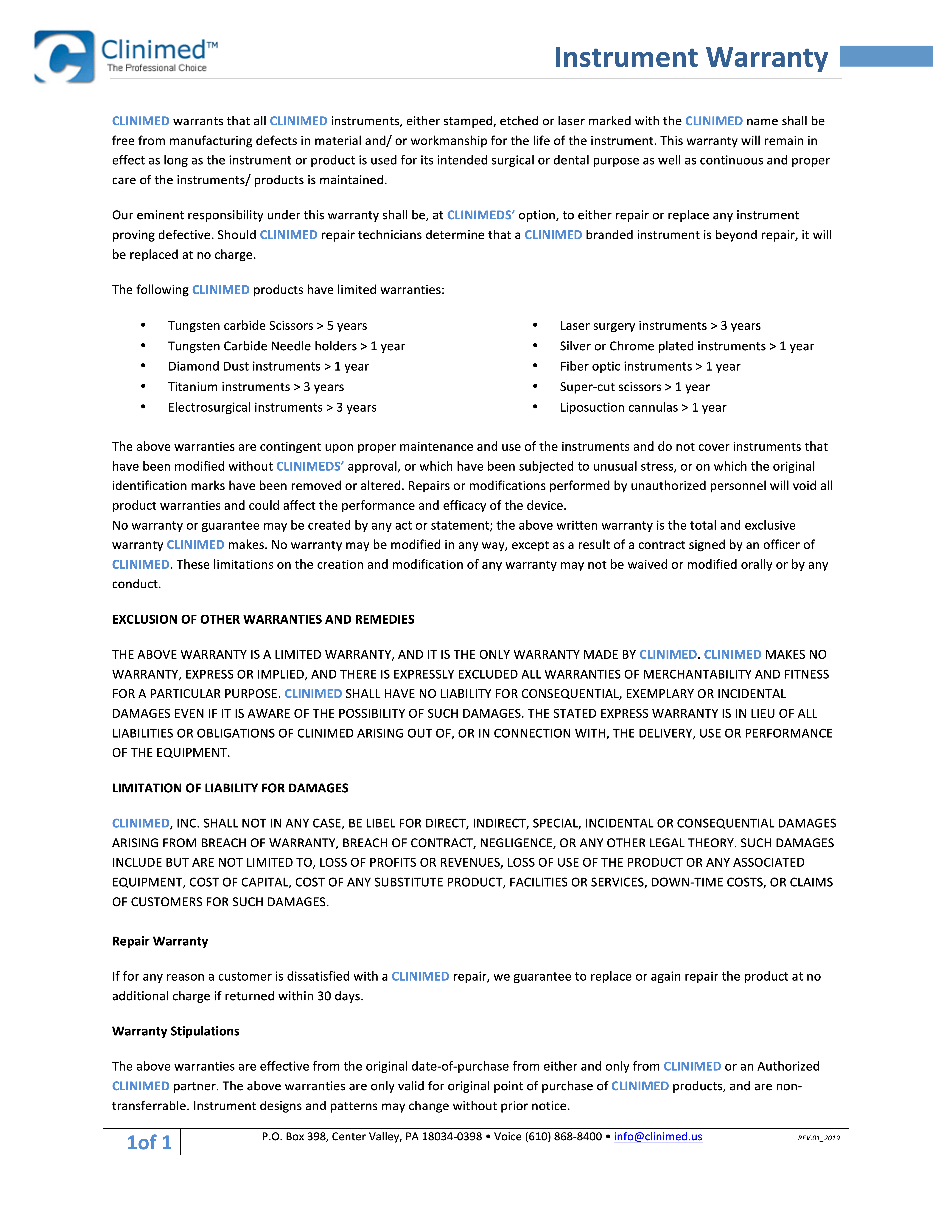In the top-left corner of the image, we see the Kleinemed trademark along with the phrase "The Professional Choice." The text details the warranty coverage for Kleinemed instruments, explaining that items stamped, etched, or laser marked with the Kleinemed name are guaranteed to be free from manufacturing defects in material and workmanship for the instrument's lifetime. This warranty is valid as long as the instrument is used for its intended surgical or dental purpose and is maintained with continuous and proper care. The warranty states that Kleinemed will either repair or replace any defective instruments at their discretion. If a Kleinemed technician determines that an instrument is beyond repair, it will be replaced free of charge. The document appears to be an official warranty statement for Kleinemed instruments.